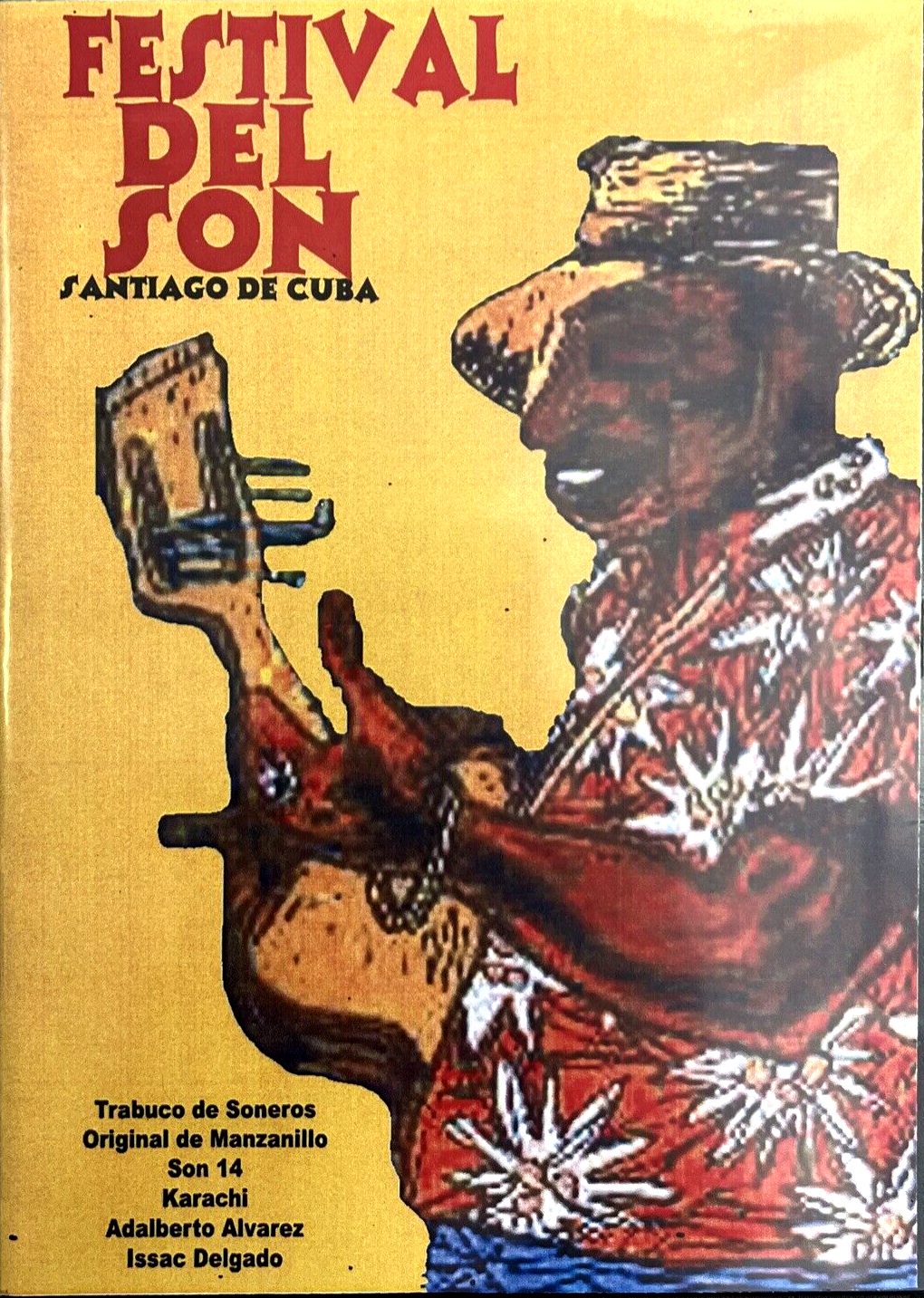This vibrant, full-color poster advertises the "Festival del Son," set to take place in Santiago de Cuba. The background is a striking yellow, with the festival name prominently displayed at the top in vertically stacked red capital letters. Below that, in black font, it reads "Santiago de Cuba." The captivating image features a man with dark skin, glowing white teeth, and a broad smile. He dons a red Hawaiian shirt adorned with white sunburst patterns, and a wide-brimmed straw hat shields his eyes. His accessories include a silver bracelet and a ring. This stylized drawing depicts the man playing a guitar. At the bottom left, the poster lists the festival's featured artists: Trabuco de los Soneros, Original de Manzanillo, Son 14, Karachi, Alberto Alvarez, and Isaac Delgado.